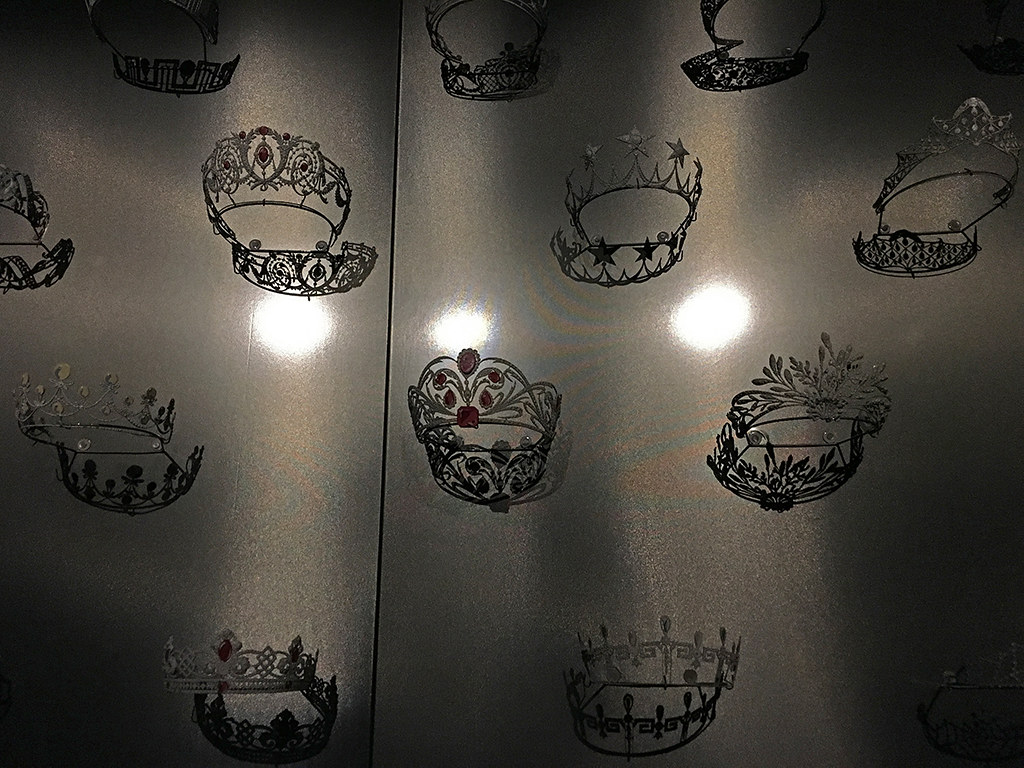This image features a highly polished cabinet with a metallic, pewter-toned surface adorned with intricate designs of royal crowns and tiaras in various styles and sizes. The cabinet is divided vertically by a black seam running about one-third from the left edge. The crowns and tiaras, embellished with jewels and distinctive shapes, are vividly highlighted against the glossy background. Three bright round lights reflect off the cabinet's surface, indicating that illumination from an external light source is casting circular highlights on it. The crowns are arranged in rows, with their intricate patterns including elements like stars, leaves, arches, and gemstones. The detailed craftsmanship and the repeated royal motifs create a sparkling, regal aesthetic on the sleek, light-gray backdrop.